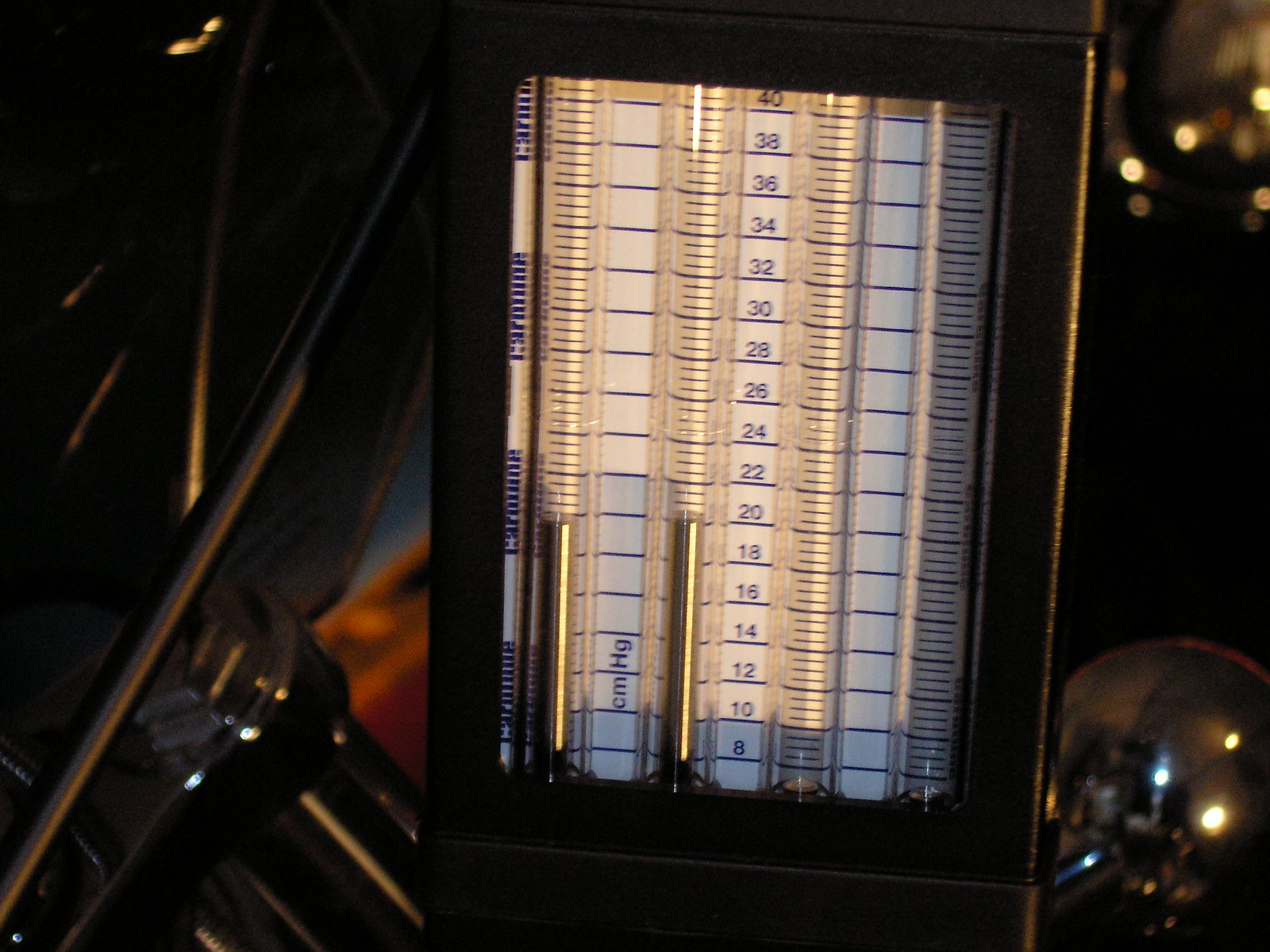The photograph is dark and poorly lit, obscuring many details. On the left side of the background, a cluster of shiny chrome metal pipes can be discerned, adding a reflective element to the otherwise shadowy scene. The right side of the background features two large, metallic spheres, contributing to the industrial ambience.

Centrally positioned in the image is a rectangular device with a metal frame. This apparatus houses three vertical thermometer-like structures. The thermometers are separated by small, white square spaces. The background behind the thermometers is white, adorned with blue grid lines forming squares. The central thermometer features a sequence of descending numbers starting from 40 at the top and decrementing by increments of two down to 8 at the bottom. This numbering system is mirrored on the two additional thermometers flanking the central one, which also display their scales prominently.

Overall, the image captures complex, industrial equipment with a focus on measurement devices that provide a precise, numerical readout within a stark, utilitarian setting.